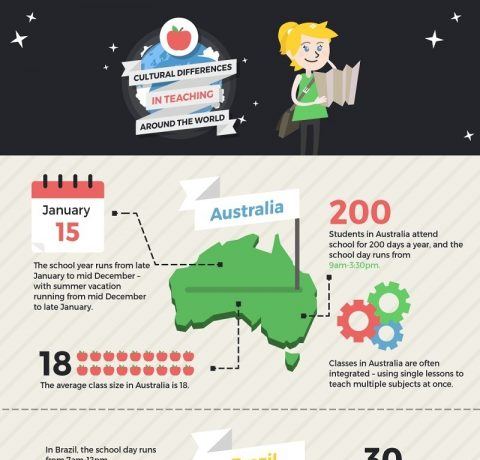The image is a detailed infographic poster titled "Cultural Differences in Teaching Around the World." At the top, there's a black banner adorned with small white stars and a circular emblem featuring a red apple atop a globe, flanked by clouds. Within this black banner, there's a white ribbon with black text that says "cultural differences in teaching" and red text reading "around the world." To the right, an illustration of a smiling girl with blonde hair, blue eyes, and white skin is depicted holding a map. She wears a green dress over black pants and carries a school or office bag slung across her shoulder.

Below the banner, the infographic continues on a beige background with subtle diagonal stripes. It prominently features a map of Australia with a small flagpole and a flag labeled "Australia." Next to the map, it states that the school year runs from late January to mid-December, with specific information pointing to January 15th as the start date and mid-December as the beginning of summer vacation. Another text box indicates that the average class size in Australia is 18, symbolized by 18 apple icons. Large red text reading "200" highlights that Australian students attend school for 200 days a year, with school days running from 9 a.m. to 3:30 p.m. Below this, there's an illustration of cogs with text detailing that classes in Australia often integrate multiple subjects into single lessons. The poster uses a color palette that includes green, red, blue, orange, black, beige, and tan.